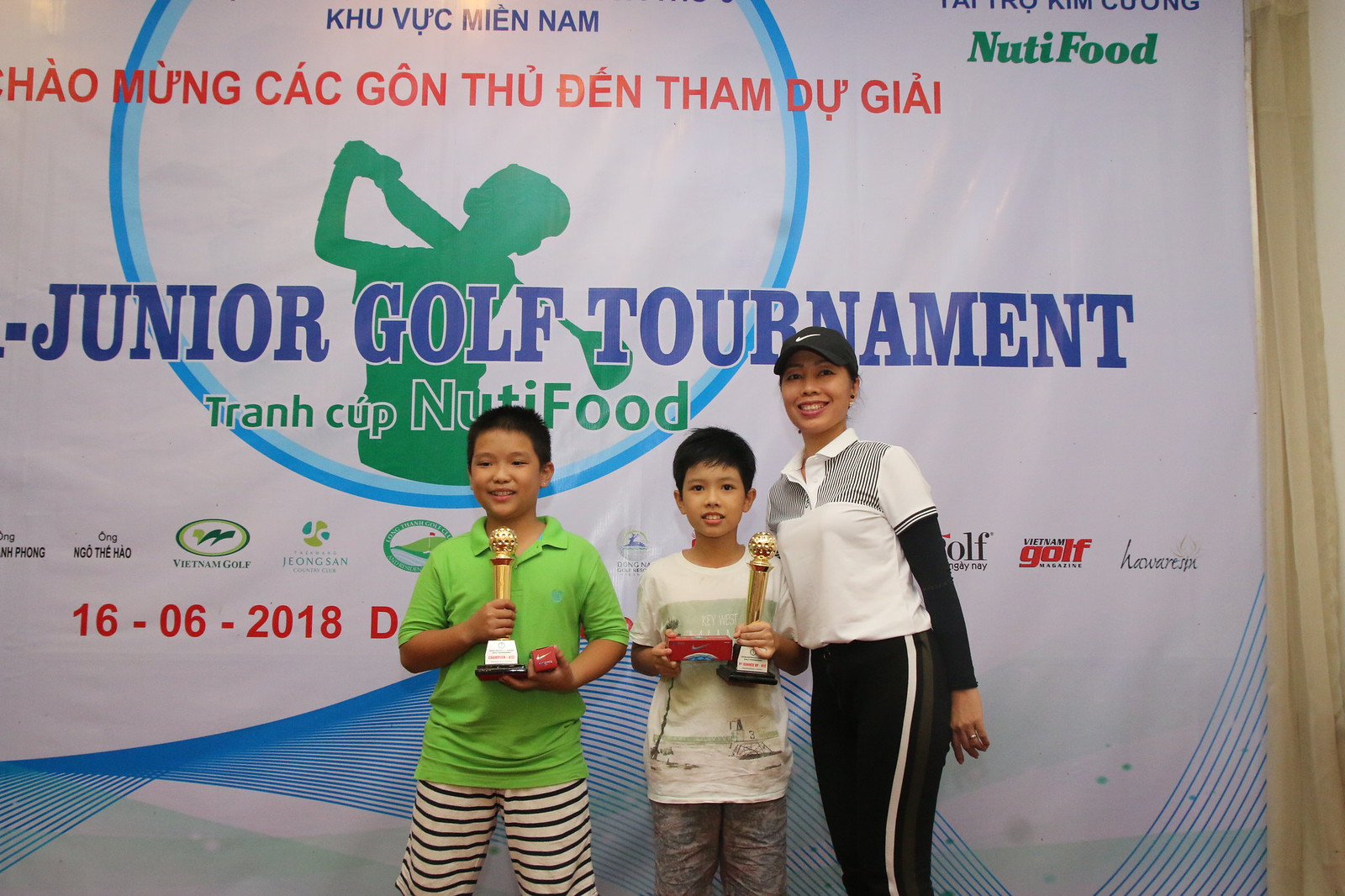In the image, two young boys stand beside a woman, likely their mother, in front of a banner announcing a Junior Golf Tournament. The banner, white with blue and red writing, includes the name "Tron Cup Nudafood," suggesting Nudafood as the primary sponsor along with other smaller logos at the bottom. The date "16-6-2018" (June 16, 2018) is noted on the left side of the image. 

Both boys, appearing to be around nine or ten years old and nearly the same height, hold tan-colored trophies. The boy on the left wears a solid green polo shirt paired with black and ivory striped shorts. His companion to the right sports a white t-shirt partially obscured by his trophy and gray shorts. 

The woman, clad in a Nike baseball cap, wears a predominantly white long-sleeve shirt with black accents and a black undershirt extending down her arms. She also sports black bottoms with a distinctive white stripe along the sides. A ring on her ring finger hints at her marital status. All three individuals are standing in a row, smiling proudly as they hold the trophies in front of the tournament banner, likely celebrating the boys' achievements in the event.